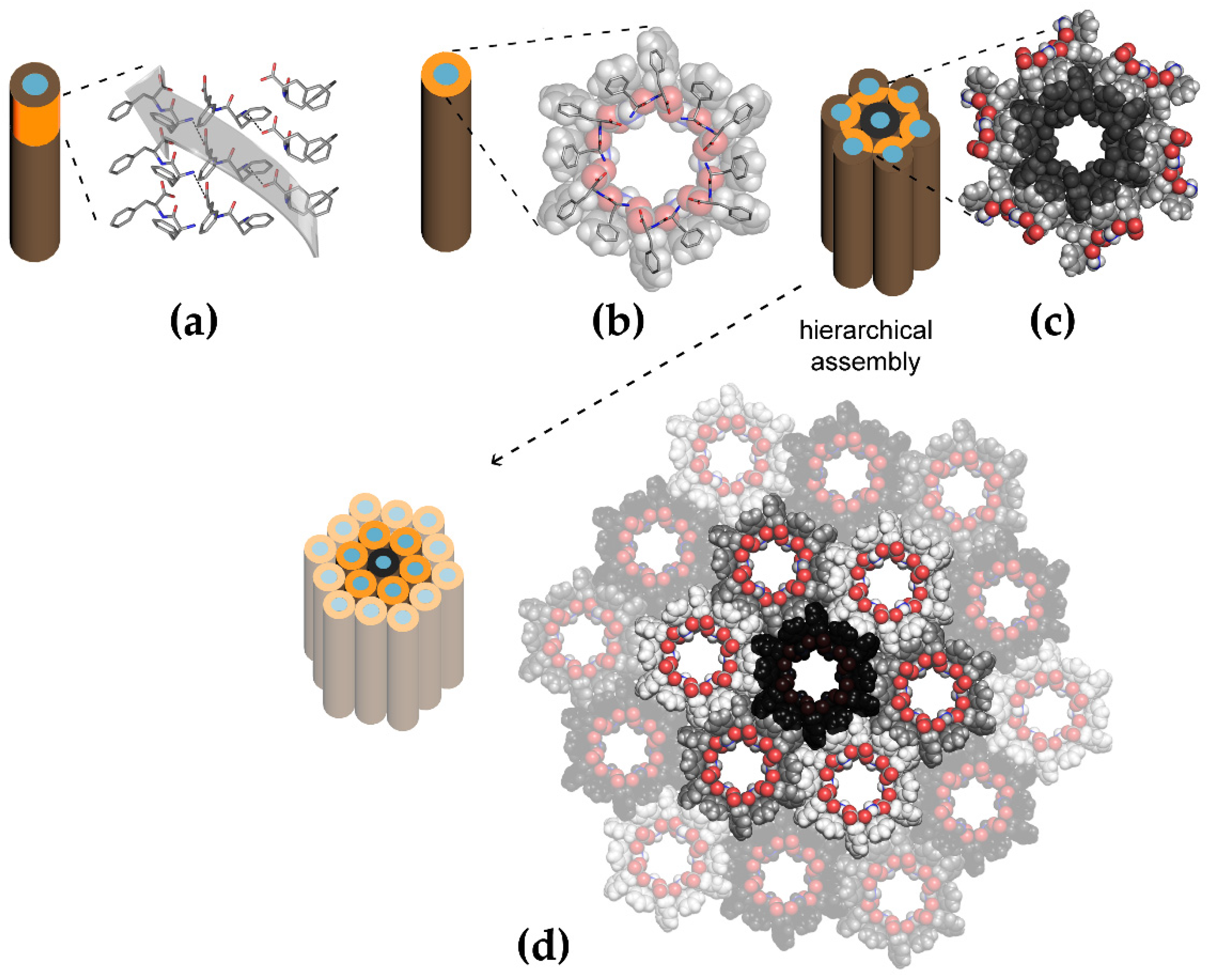The image is a scientific diagram showcasing the hierarchical assembly of molecular structures. The background is white and prominently features parts labeled A, B, C, and D in lowercase parentheses. 

In Part A, there is a brown, battery-shaped object with a blue center, surrounded by yellow regions. Dotted lines extend to the right, connecting to a gray ribbon-like entity alongside scattered molecules.

Part B mirrors the components of Part A with the brown, battery-shaped structure and dotted lines. However, the molecules have now assembled into a wreath-like formation—gray with a red core.

Part C advances this theme; the battery shapes have multiplied into a ring, emphasizing the process of hierarchical assembly. The molecular wreath from Part B has become larger, now featuring a black center. Dotted lines lead downward to Part D.

In Part D, the diagram shows an expansive multiplication of the battery shapes and wreath elements seen in Part C. The wreaths are now numerous, with a black core in the middle, encircled by both a solid and a transparent ring of molecules, indicating a further level of organized complexity.

Overall, the image is brightly lit and clear, giving an in-depth view of molecular assembly processes, emphasizing how smaller structures integrate into larger, complex formations.